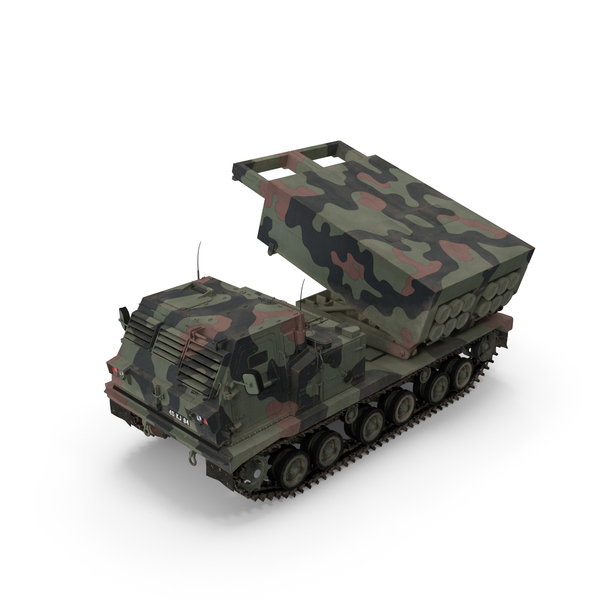The image depicts a toy military vehicle inspired by a real design. Set against a completely white background, the vehicle is positioned diagonally with its shadow extending towards the 7 o'clock direction. The toy features a rectangular and square trapezoid shape with camouflage colors—including dark green, black, brown, and light pink patterns. Equipped with tank treads and six tires, it closely resembles a tracked military tank. The vehicle has an armored front section with slitted viewing ports, vents, a door with a window and a mirror, as well as some indistinct numbers or text printed on it.

Prominently, the back of the toy features a turreted section that houses a grid of 12 missile launchers, capable of being raised and rotated to various angles. This section is shoebox-shaped, and the missiles are vividly detailed, appearing like small circles from certain angles. Despite its simple design, the toy is accentuated with antennas and various exposed details, adding to its resemblance to an actual military vehicle. The combination of imaginative design, accurate colors, and practical details make it an intriguing and dynamic model that captures the essence of a missile-launching tank.